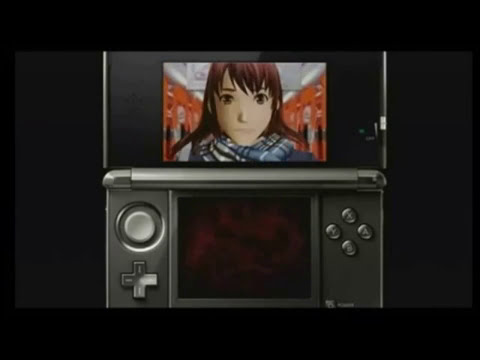The image showcases a silver, handheld Nintendo DS video game system against a completely black background. The device is opened, revealing two screens: the top screen, surrounded by a black bezel, displays a close-up of an animated female character with long brown hair and bangs, wearing a blue, black, and gray checkered scarf, and standing in what seems to be a school hallway with orange lockers on either side. The bottom screen is currently blank. The control layout features a cross-shaped directional pad and a joystick on the left side, along with four round buttons (Y, X, A, B) arranged in a diamond pattern on the right. It looks like a modern interpretation of a classic handheld gaming device, captured in a close-up photograph with no visible hands holding the unit.